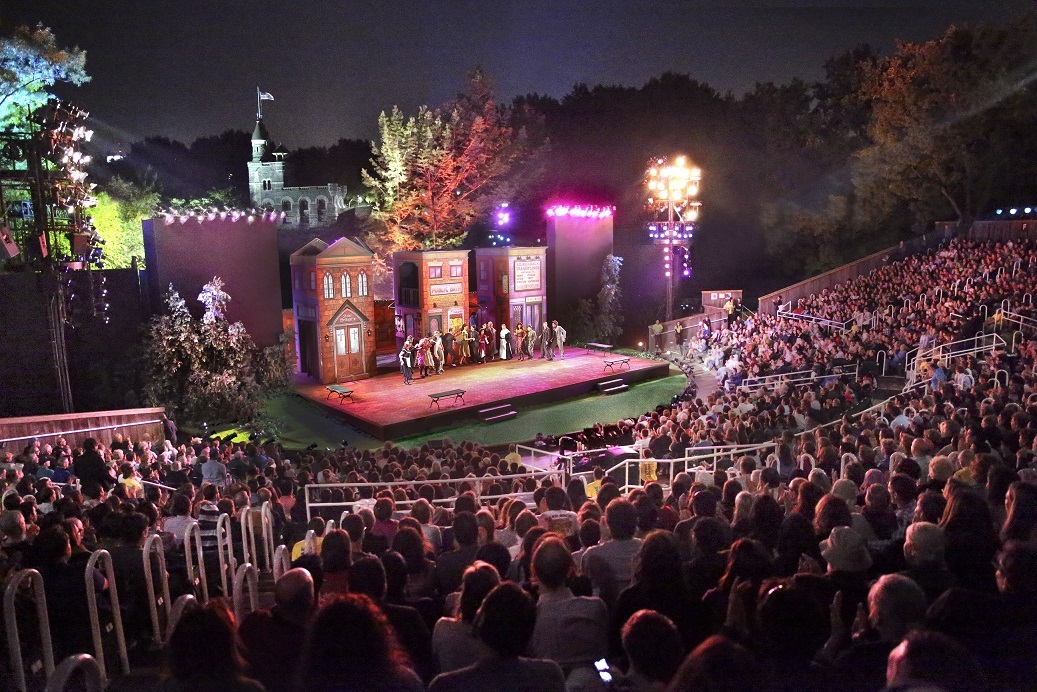This professional nighttime color photograph captures a lively performance in a crowded outdoor amphitheater with semi-circular seating. The amphitheater, full with approximately 300 spectators, stretches from the bottom of the stage up into higher risers towards the back. The well-lit stage is approximately 40 feet wide by 20 feet deep and features a setup resembling three turn-of-the-century townhouses side-by-side with small gaps between them. Twelve performers, dressed in medieval or turn-of-the-century period clothing, animate the scene under the glow of large clusters of lights mounted on metal poles. On either side of the stage, forest-like surroundings and trees showing fall colors frame the performance area. In the far background, a castle backdrop enhances the visual depth, suggesting a theatrical performance possibly within an amusement park setting. The clear night sky, devoid of stars, blankets the entire scene, while light jackets on the audience hint at a cool autumn evening.